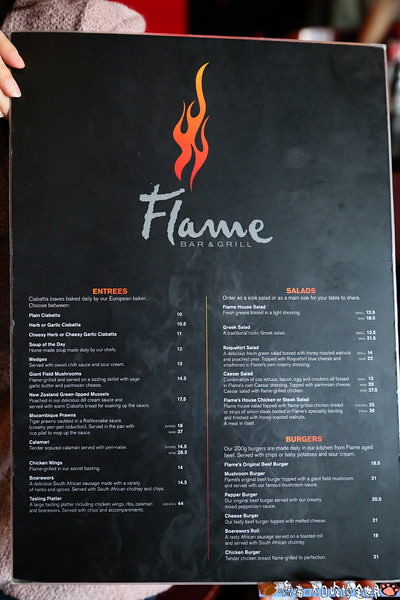This photograph captures a menu from a restaurant called Flame, presented against a black background. The menu itself is rectangular and is held vertically by a hand visible on the right side and part of a red and white sweater on the left. At the top center of the menu, a flame design is prominently displayed, colored in vibrant shades of red and orange, ascending towards the top edge. Below the flame icon, the word "Flame" is printed in gray, followed by "Bar and Grill" in block letters in the same color.

The left section of the menu lists entrees, highlighted in red font, while the right section features options for salads and burgers, also printed in red block letters. At the very bottom of the menu, there is some blue text, which appears illegible in the photograph.

The hand holding the menu has light skin, with well-manicured fingernails, and three fingers are visible clutching the edge of the menu, pointing downwards towards the right. Additionally, portions of the red and white sweater are visible both in the upper left and bottom left corners of the image.